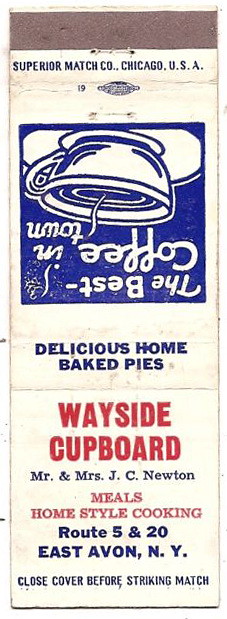This detailed matchbook design displays a vintage advertisement for Wayside Cupboard. The cover features a striking strip at the top, with "Superior Match Company, Chicago, USA" inscribed below it. A prominent illustration of a coffee cup with steam rising, accompanied by the slogan, "The Best Coffee in Town," dominates the center section. Below this image, text in blue reads, "Delicious Home Baked Pies." The lower part of the matchbook is emblazoned with the name "Wayside Cupboard" in vivid red, followed by "Mr. and Mrs. J.C. Newton" in smaller red font. The phrase "Meals Home Style Cooking" appears next, also in red, with the location specified as "Route 5 and 20, East Avon, New York" in blue text. The instruction "Close cover before striking match" is printed at the bottom, ensuring safety. The background is predominantly white, with blue accents and red highlights, giving the overall design a nostalgic and homey feel.